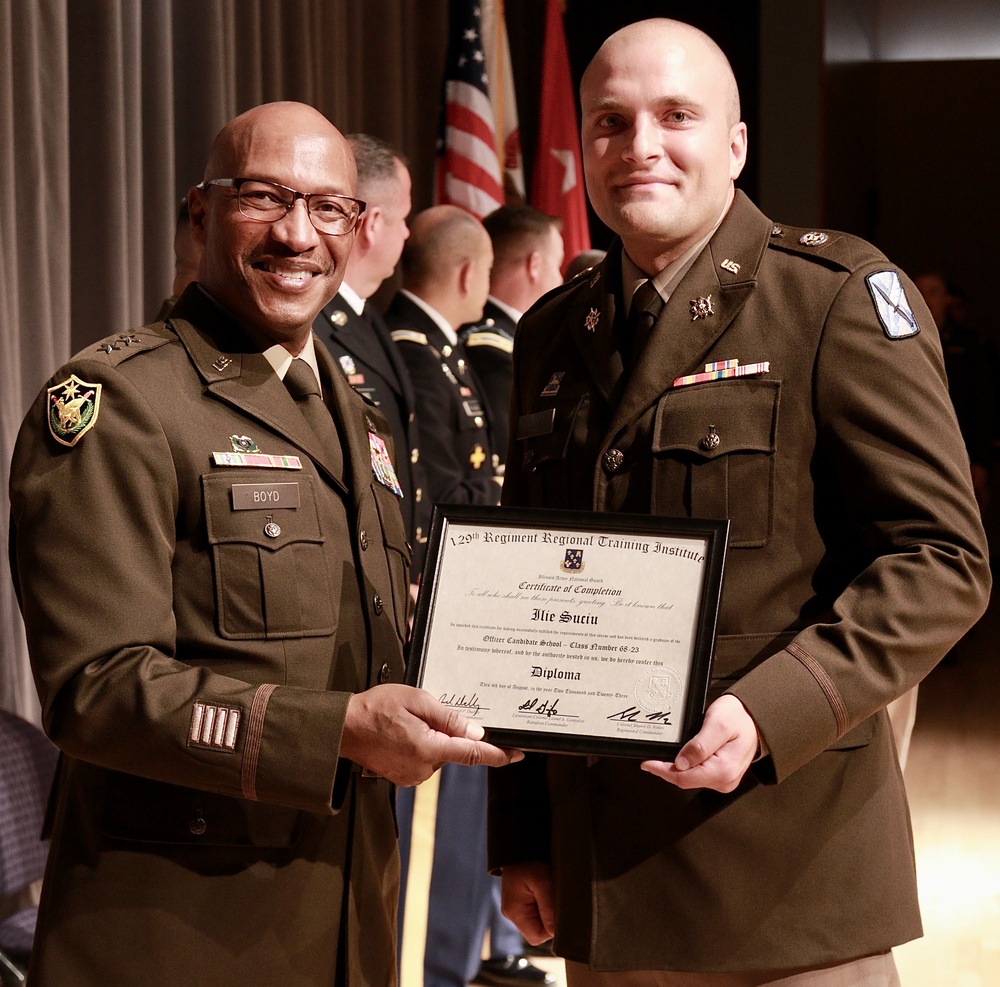In this professional color photograph, two military men dressed in formal uniforms are prominently featured on a stage with a gray curtain in the background. Both men, a friendly-looking older Black gentleman with glasses and a bald head named Boyd, identified by his name tag, and a younger bald White man in his 20s or 30s, are holding up a black-framed diploma or certificate from a Regional Training Institute, signifying the completion of a training program. Their uniforms, adorned with various emblems, pins, and patches—including a notable star and bird patch on Boyd's right shoulder—exhibit shades of brown, dark green, and gray. The setting is further accented by the presence of an American flag and another flag consisting of red, white, and blue colors. Three other military personnel are visible in the background, contributing to what appears to be a ceremonial or graduation event marked by professionalism and pride.